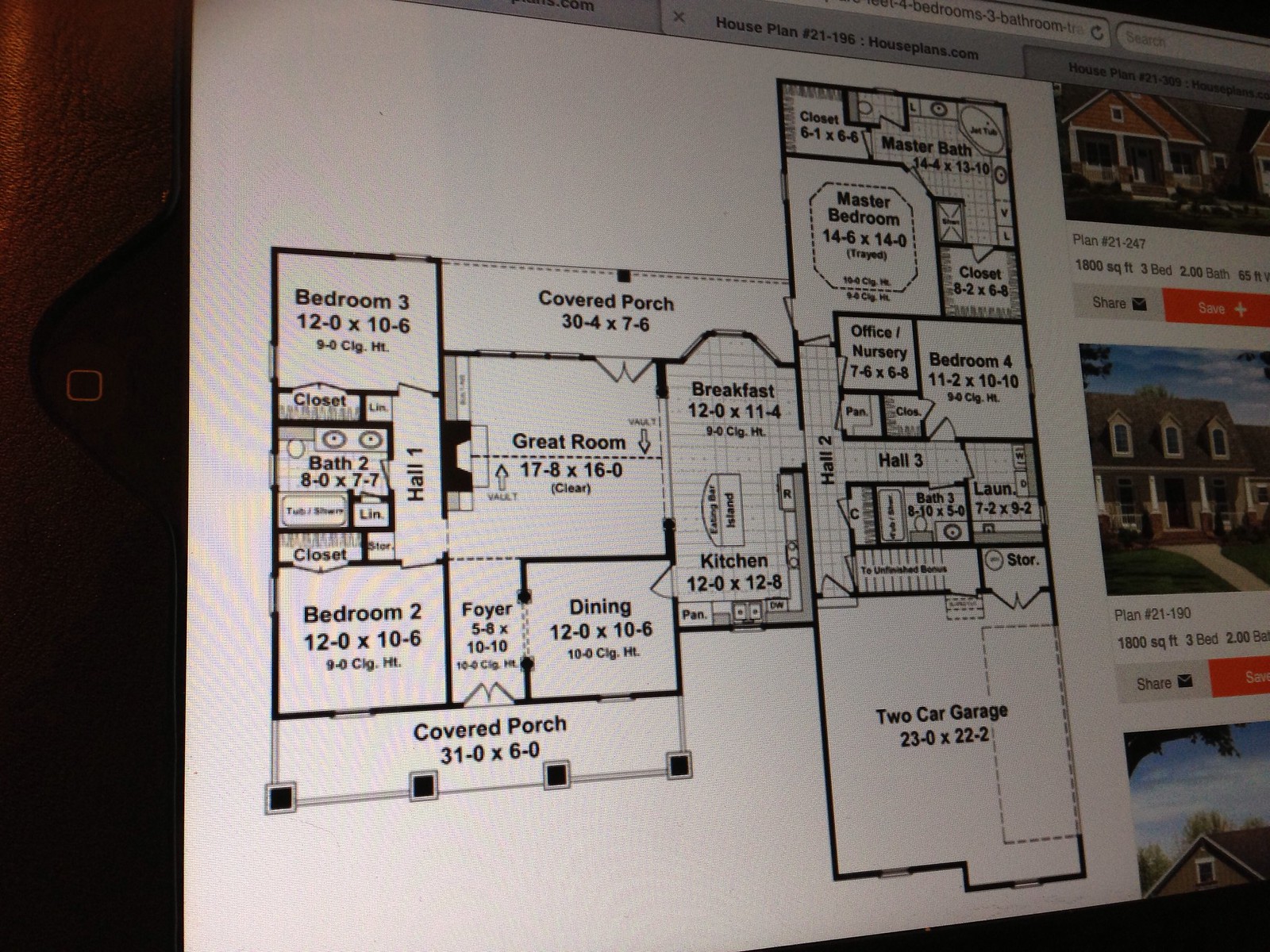The image captures a highly detailed blueprint of a house displayed on a computer screen. The screen is part of a large rectangular setup that reveals a digital layout, with a backdrop featuring a gray wall and a black object outlined by a yellow square to the far left. The blueprint itself intricately maps out various sections of the house, including a two-car garage, covered porch, bedrooms, office, and nursery, complete with sizes and locations clearly marked. Accompanying the blueprint on the screen are pictures of houses sourced from a website, providing additional details such as square footage and the number of bathrooms and bedrooms. On the right side of the screen, there are actionable buttons, like a gray button labeled "Share" and another labeled "Save." Multiple open tabs with close (X) icons are visible, allowing spatial organization and easy switching between different house plans. At the top, the web address and search bar are clearly displayed, reflecting the online nature of this house plan exploration.